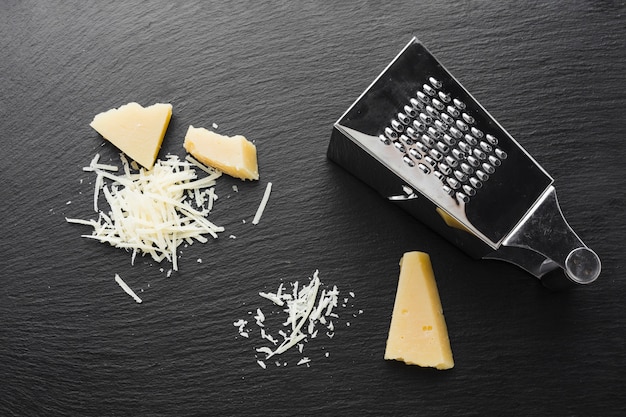The image depicts a dark brown wooden table with a distinctive metal cheese grater standing toward the right side. The cheese grater is the traditional type that can be held from the top and features openings for grating on its sides. Surrounding the grater are three large wedges of Parmesan cheese, suggesting they have been partially grated as evidenced by a few shreds stuck in the grater itself. Additionally, the table holds two small piles of freshly grated Parmesan cheese positioned off to the left. The scattered and chunkier pieces of cheese add to the impression that some active grating has recently taken place. The scene is devoid of any people, entirely focusing on the grated and whole cheese amidst the rustic wooden tabletop setting.